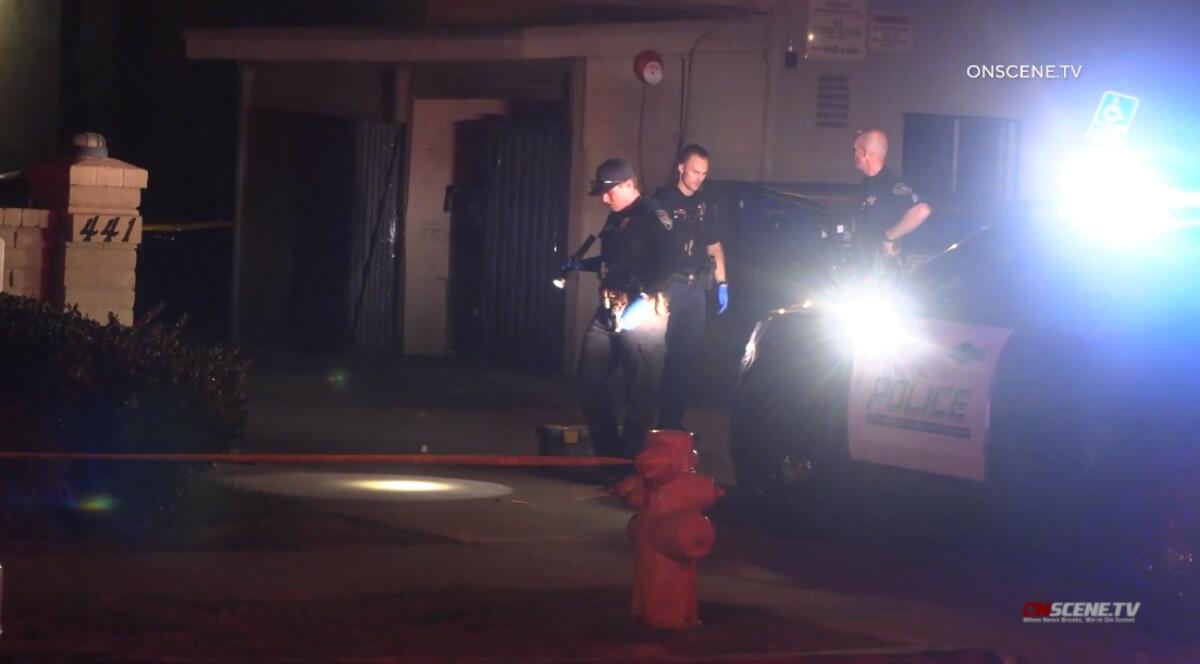The image captures a night scene of police investigating an incident outside an entrance, likely to a business or residential building. Three officers, dressed in black uniforms and some wearing blue rubber gloves, are positioned near a police car with its top lights flashing blue and white, illuminating the area. One officer stands to the left, focused downward, shining a flashlight onto the concrete sidewalk, possibly searching for evidence. Behind him, two other officers engage in conversation. Prominent in the foreground is a red fire hydrant wrapped with red tape. Adjacent to this, a white brick pillar marked with the number 441 stands against the structure. The background reveals an industrial dumpster and a fire alarm affixed to the building. The scene is marked with the logos "on scene dot TV" on both the upper and lower right corners of the image.